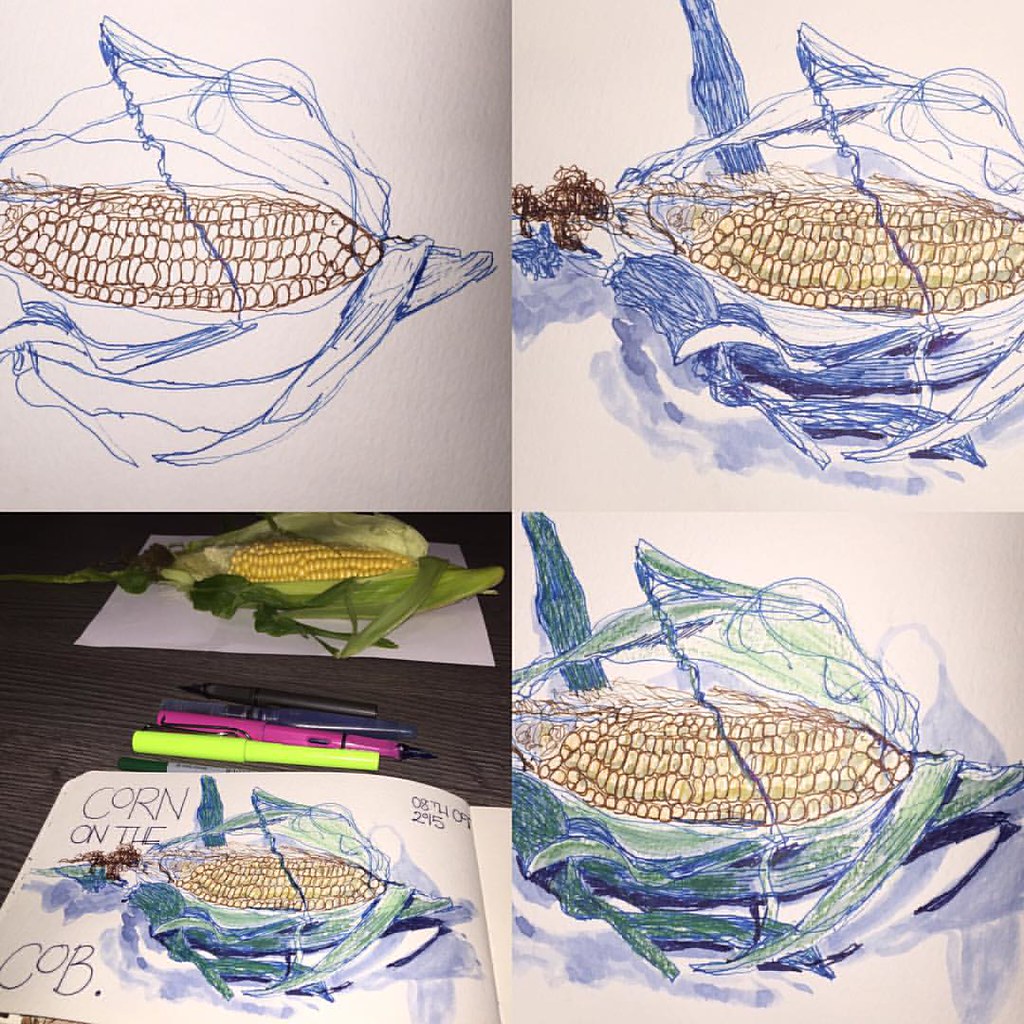The image is divided into four quadrants, each showcasing different stages and elements of a corn on the cob illustration. 

In the upper left quadrant, a detailed drawing of corn in the process of coloring is visible, outlined in blue against a white surface. The upper right quadrant features the same corn image, now with kernels shaded in light yellow while the husks remain blue. 

The bottom right quadrant reveals the completed illustration, where the green and dark green husks complement the yellow kernels in a fully colored-in corn depiction. 

The bottom left quadrant, zoomed out, shows a page from a sketchbook labeled "corn on the cob." A collection of art supplies, including a yellow highlighter, pink highlighter, blue pen, black pen, and green marker, is scattered around. Additionally, an actual corn on the cob with green and brown husks lies on a white piece of paper, contrasting with the illustrations.